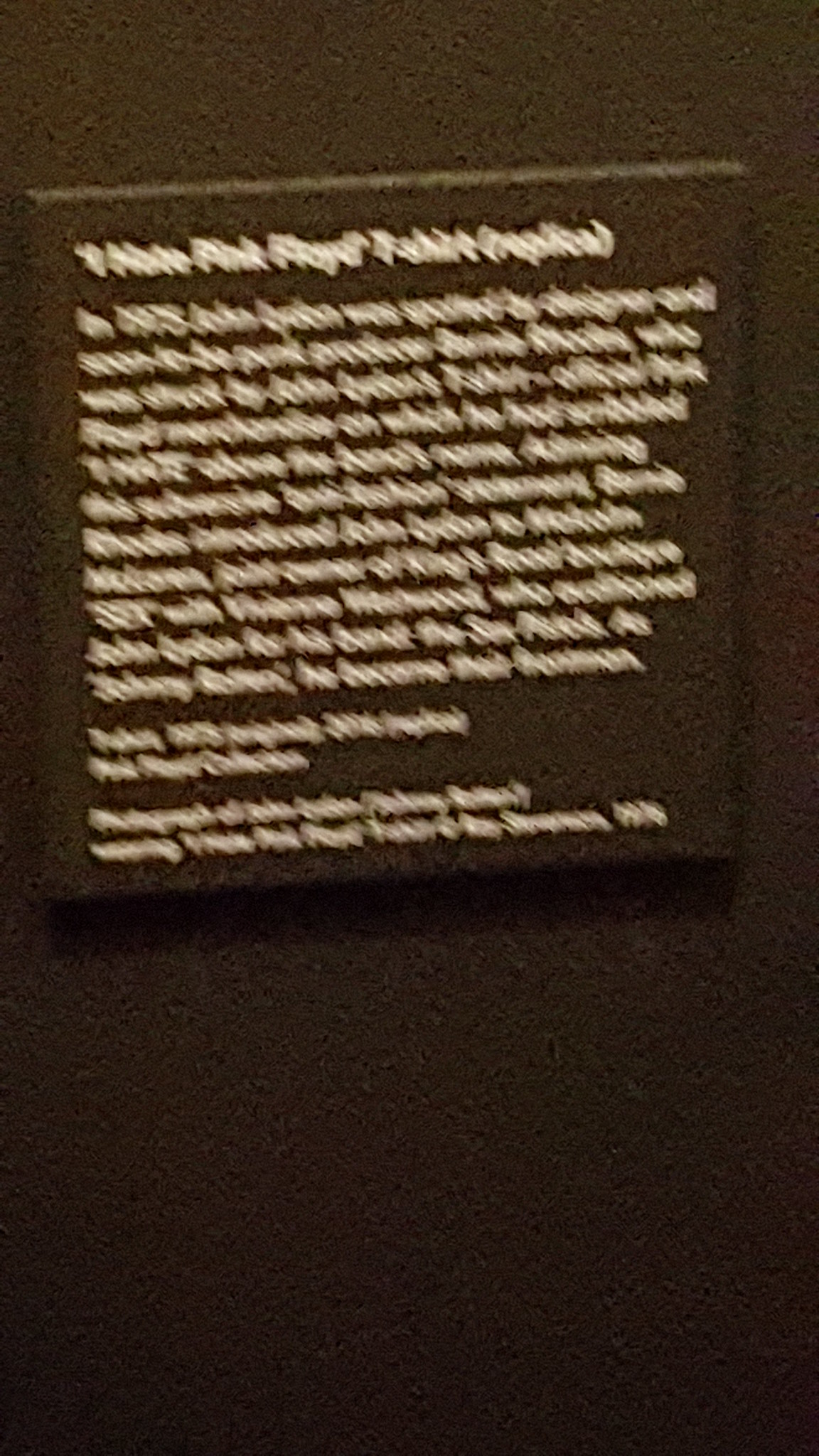This photograph captures a brown, square, raised plaque mounted on a brown stone surface. The plaque, featuring white engraved text, is quite blurry due to motion, making it difficult to discern most of the wording. However, the bold text at the top possibly reads, "I hate Pink Floyd T-Shirt Replica," with "Replica" in parentheses. Below this heading, there appears to be a detailed, yet unreadable, paragraph. Partial and blurry phrases include mentions of the years 1975 and 1978, John (Blurr's name), Buddy Rhodes, official Pink Floyd merchandise, and possibly an introduction of John Lydon to Malcolm McLaren, co-founder of The Sex Pistols. The plaque seems to elaborate on a historical anecdote regarding Pink Floyd and The Sex Pistols connection.